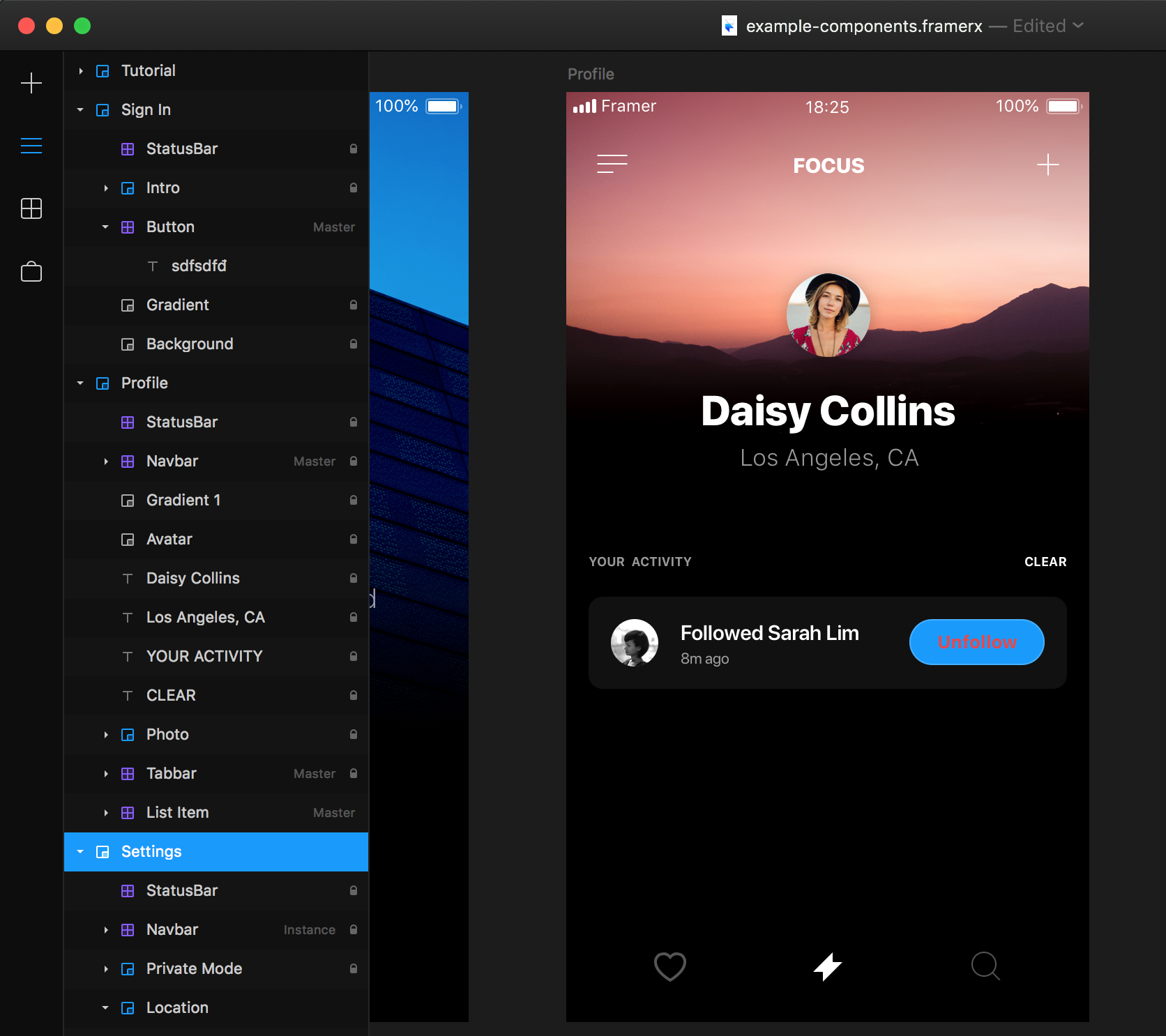Screenshot of a computer interface with a black background and various clickable options on the left-hand side. Dominating the right side of the screen, slightly off-center, is a user profile section. The header features a striking red-pink sky as the background, with a small profile photo of a girl with short, shoulder-length hair that is both brown and blonde, and she is wearing a hat. 

Her name, "Daisy Collins," is prominently displayed in large white text. Beneath her bolded name, "Los Angeles, CA" is written in smaller, unbolded white font. Below this, a section titled "Your Activity" includes a secondary, smaller black-and-white profile photo. 

Text in bold white font reads "Followed by Sarah Lim," with "8M ago" indicating the activity occurred eight minutes prior, displayed in smaller, unbolded white text. An "Unfollow" button is placed in a blue box with pink font, completing the profile summary.